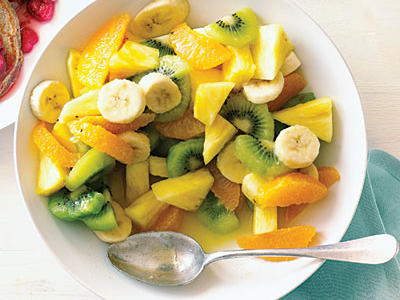This vibrant photograph, likely taken indoors, features a top-down shot of a white bowl filled with an assortment of sliced fruits, including strawberries, kiwis, pineapples, and a few orange slices nestled towards the bottom right of the bowl. Resting in the bowl is a silver spoon, hinting at the delicious freshness waiting to be enjoyed. The bowl is placed on a lightly-colored wooden table, partially covered by a teal green tablecloth visible at the bottom right corner of the image. In the top left corner, a white plate, mostly cropped out, seems to hold a stack of pancakes adorned with sliced strawberries, adding a complementary note to the scene. The meticulous arrangement and vivid colors of the fruit demonstrate a delightful, appetizing presentation.